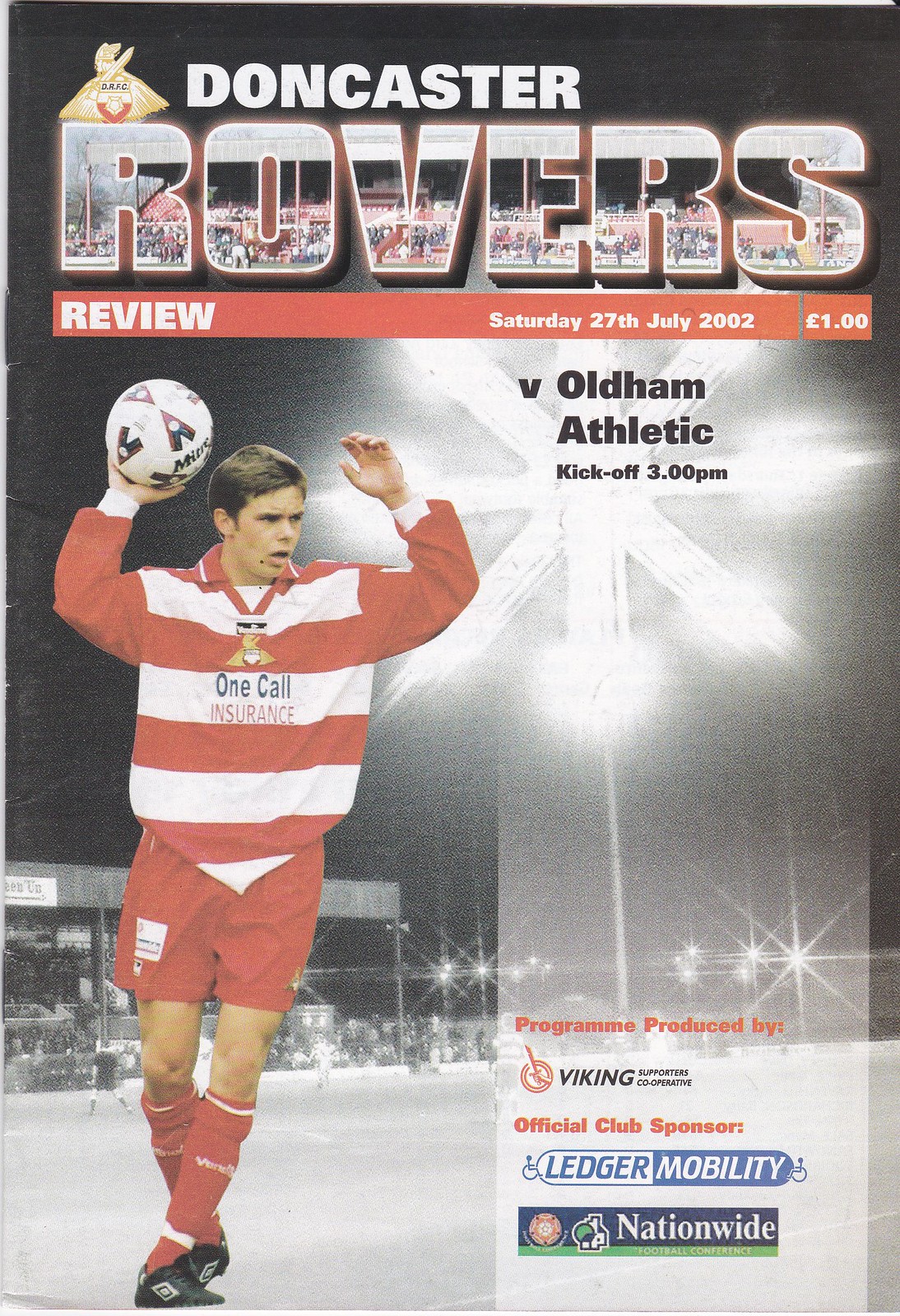The image is the front cover of a review magazine for the Doncaster Rovers soccer club, titled "Doncaster Rovers Review," dated Saturday, 27th July 2002. Dominating the left-hand side is a large, imposing image of a Caucasian gentleman clad in the team's red and white thick-striped attire, emblazoned with "OneQual Insurance" across the chest. He stands confidently with one leg crossed over the other and both hands raised, his left hand holding a white soccer ball with black writing. The player is dressed in matching red shorts, red and white striped socks, and cleats.

The scene appears to be superimposed onto a soccer field under night-time illumination, as spotlights are visible in the background along with a section of the audience to the left. At the top of the page, above the player, the text reads "Doncaster Rovers Review" followed by "Saturday 27th July 2002," indicating the publication date. The bottom of the cover features several sponsor logos, including "Programmed Product by Viking," "Official Club Sponsor," "Ledger Mobility," and "Nationwide." The overall design and layout suggest it serves to provide fans with insights and updates about their team.